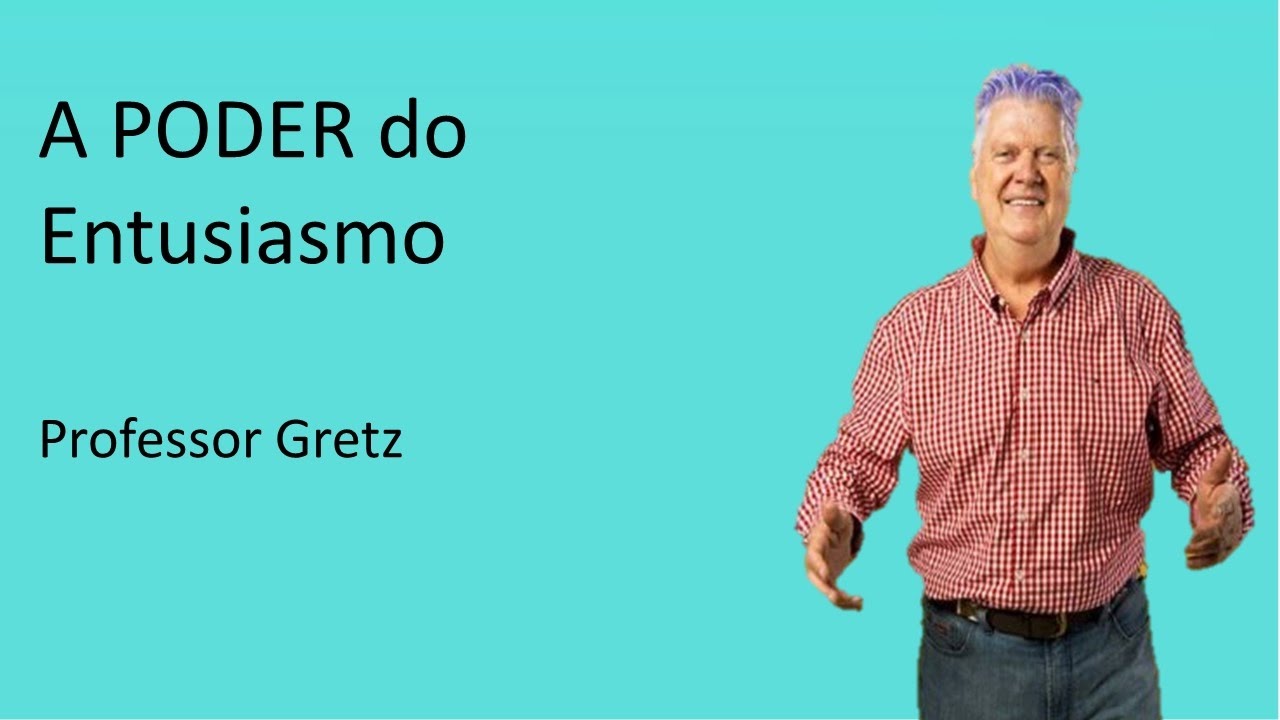The rectangular image features a bright turquoise background. On the left-hand side, in black text, is the phrase "Poder do Entusiasmo," with "Poder" capitalized. Directly below, the words "Professor Gretz" are also written in black. The right side of the image showcases a man identified as Professor Gretz, visible from just below his waist to the top of his head. He is dressed in blue jeans with a black belt and a red and white checked button-down shirt, which is buttoned up to his neck except for the top button. Professor Gretz has vibrant purple hair and is smiling broadly. His arms are outstretched with open hands, creating a welcoming and enthusiastic posture.